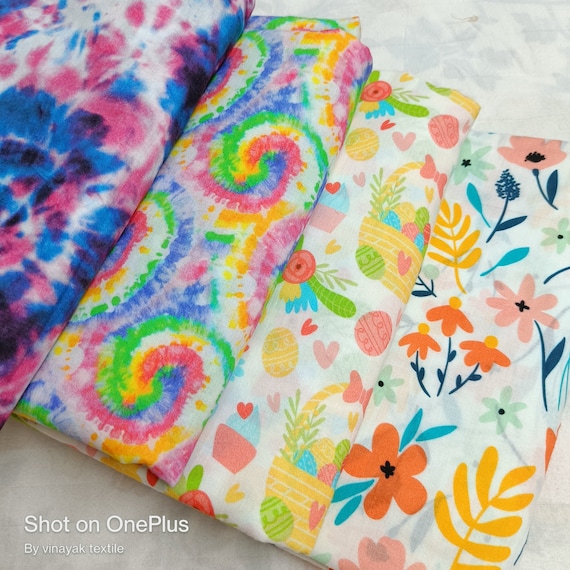This image showcases four vibrant rolls of textile fabric laid out on a white background with a faint gray floral pattern. From left to right, the first roll features a tie-dyed pattern in white, blue, and pink. The second roll also employs a tie-dyed technique, creating a swirling design of pink, green, yellow, and white. The third roll presents a charming Easter-themed print, complete with baskets of eggs, scattered Easter eggs, flowers, and hearts. The final roll on the far right displays a white background adorned with stylized, primitive-style flowers, including a daisy marked with a cross and clusters of orange flowers with yellow centers, interspersed with leaves. In the lower left corner, white text reads "Shot on OnePlus by Vignac Textile," signifying the origin and method of the photograph.